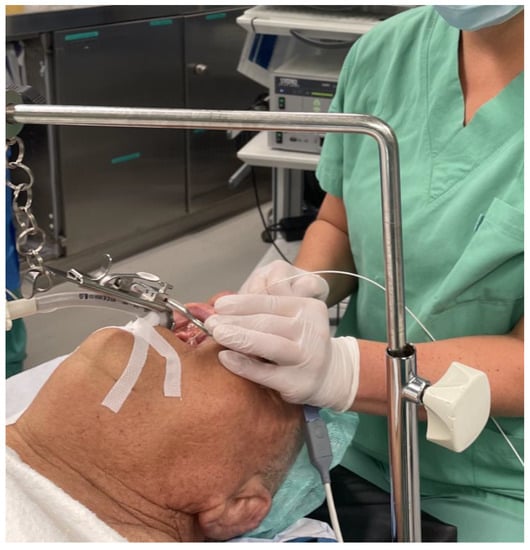The image portrays a medical or dental procedure involving an older man lying on a hospital bed. His mouth is open and obscured by a tube, which is taped to his chin. The tube is likely part of a medical device, which is being attended to by a healthcare professional. The professional, whose face is partially obscured by a light blue surgical mask, is wearing teal-colored scrubs and opaque white surgical gloves. Her hands are positioned over the man's face, working on the device in his mouth. Visible in the background are stainless steel cabinets with teal green labels or markings. A metal bar frame, possibly for medical purposes, arches over the bed, and there's a white handle attached to the frame on the left side. The overall scene is cluttered with hoses and wires, contributing to an unsettling atmosphere.